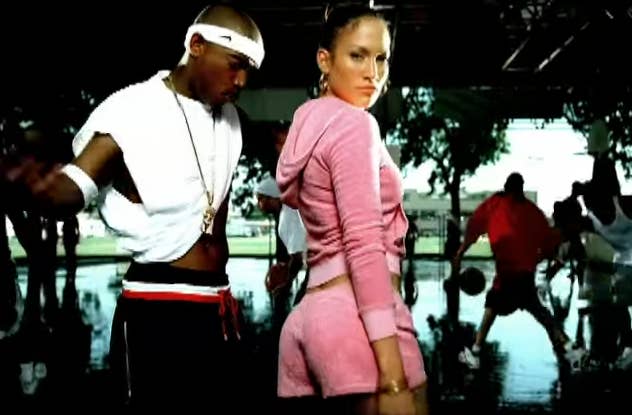This detailed image is a screenshot from a music video featuring Ja Rule and Jennifer Lopez (J-Lo). In the center, J-Lo stands wearing a pink velvet tracksuit, consisting of a long-sleeved hoodie and matching shorts that reveal part of her midriff. Her dark hair frames her face, adorned with hoop earrings and a couple of gold bracelets on her right wrist. Her head is turned slightly towards the camera, capturing a side view of her profile.

Next to her, on the left, stands Ja Rule, characterized by his bald head and a white headband. He sports a white muscle tank that shows a glimpse of his stomach and an armband on his right arm. He accessorizes with a necklace hanging over his shirt and dark shorts with a red, white, and black-striped waistband.

In the background, the scene broadens to an outdoor setting with a shiny surface and people engaged in a basketball game. Further in the distance, there's water, possibly a lake, flanked by grass and a few buildings. Visible amid the background are a few trees, some people under a cabana, and a larger man potentially working out with weights. The sky above completes this vibrant and dynamic scene from their music video.